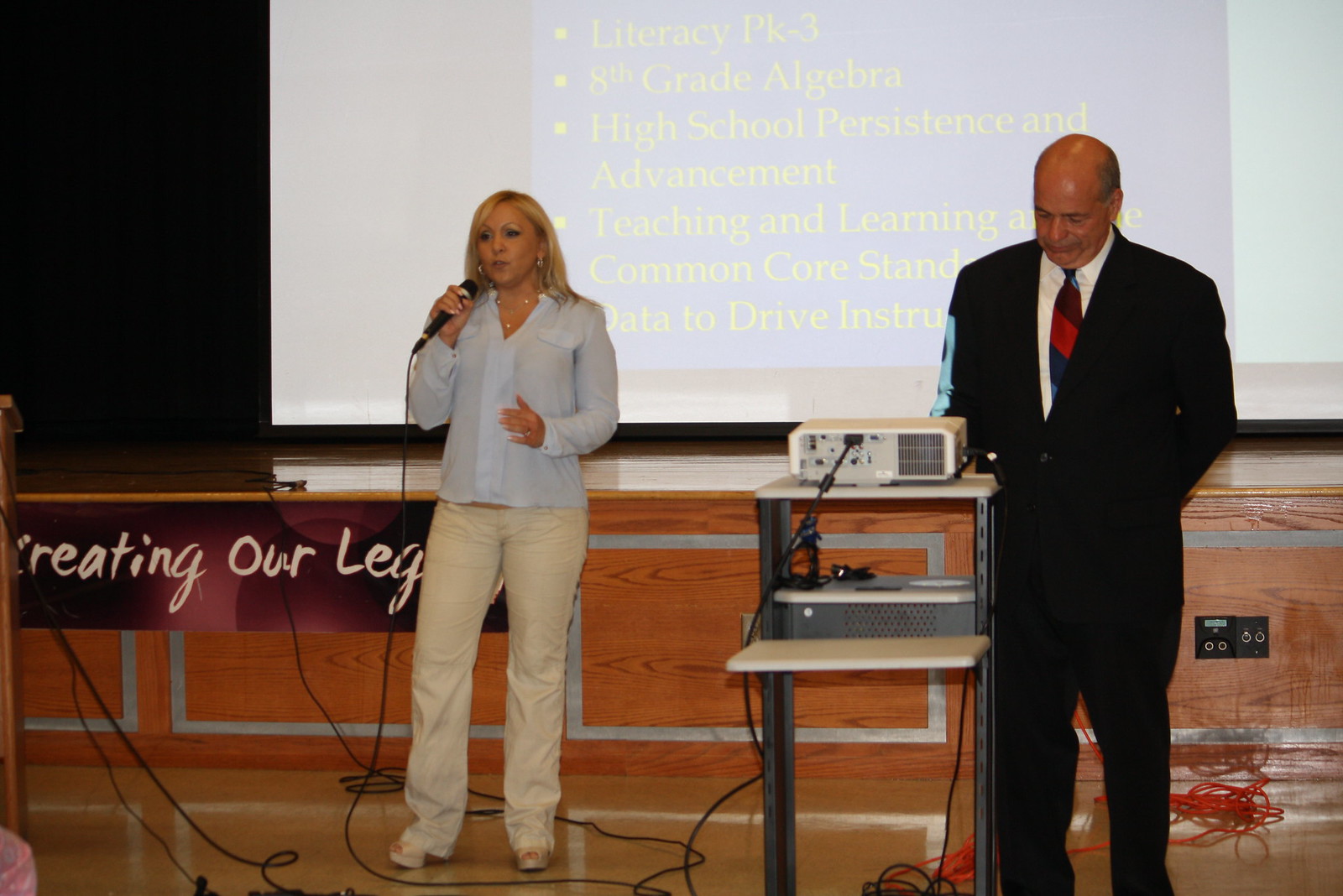In the image, an older man and a middle-aged woman are standing on a stage, likely in a school auditorium, giving a presentation. The man, approximately in his late 50s or early 60s, is dressed in a black suit with a white shirt and a red and black striped tie. He is balding on top with short hair on the sides and appears to be operating a projector positioned in front of him. The projector displays a screen behind them with educational topics such as "Literacy Pre-K to 3," "8th Grade Algebra," "High School Persistence and Advancement," "Teaching and Learning," "Common Core Standards," and "Data to Drive Instructions."

The woman, in her 40s, is standing to the left of the man. She has blonde hair, wears makeup, and is clad in a blue long-sleeved Oxford shirt, beige pants, and beige heels. She is holding a black microphone and is adorned with a gold necklace featuring pearls. Behind her is a prominent sign reading "Creating Our Legacy," set against wood grain paneling with silver squares.

The stage is equipped with numerous red and black wires that are connected to the projector and other equipment. The scene depicts an ongoing seminar focused on various educational initiatives aimed at enhancing teaching and learning methodologies.